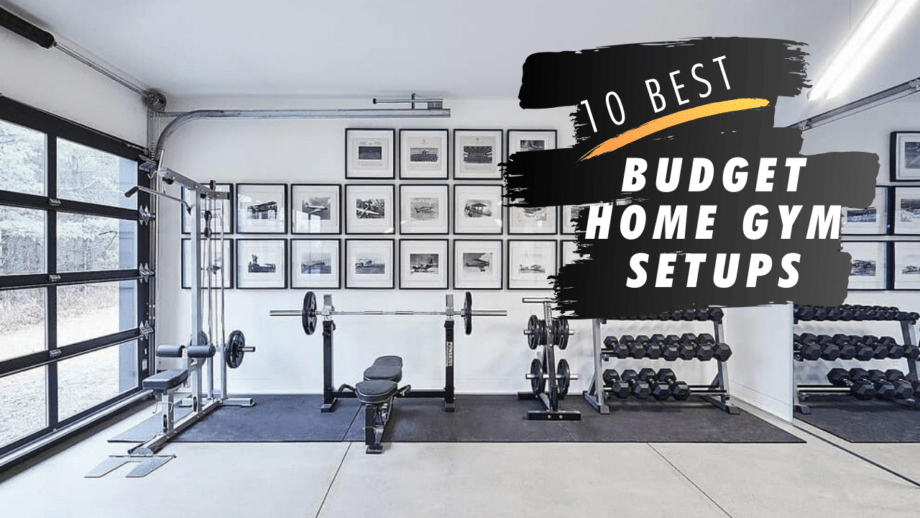In the photo, a tidy and brightly lit home gym setup is depicted within a garage space. The gym features a number of key pieces of exercise equipment: a bench press, a leg press machine, a pull-down machine with a bar, and a variety of free weights, including an array of dumbbells organized neatly on a rack. The equipment is placed on a dark rubber mat, providing a dedicated, secure workout area. The gym boasts white walls and a smooth, white ceiling, creating a pristine atmosphere. There is a see-through garage door with black frames, allowing ample natural light to flood in, complemented by fluorescent lighting on the walls. A large mirror is affixed to one side of the room, aiding in form checks during workouts. The far wall, painted white, is adorned with a series of equally spaced black-and-white photographs framed in black, adding a touch of personalization and inspiration. Prominently displayed in bold white text on a black background in the right-hand corner of the screen, the title "10 Best Budget Home Gym Setups" indicates that the image is part of a guide on how to create an effective home gym on a budget, most likely aiming to inspire and instruct viewers on assembling similar setups in their own garages.